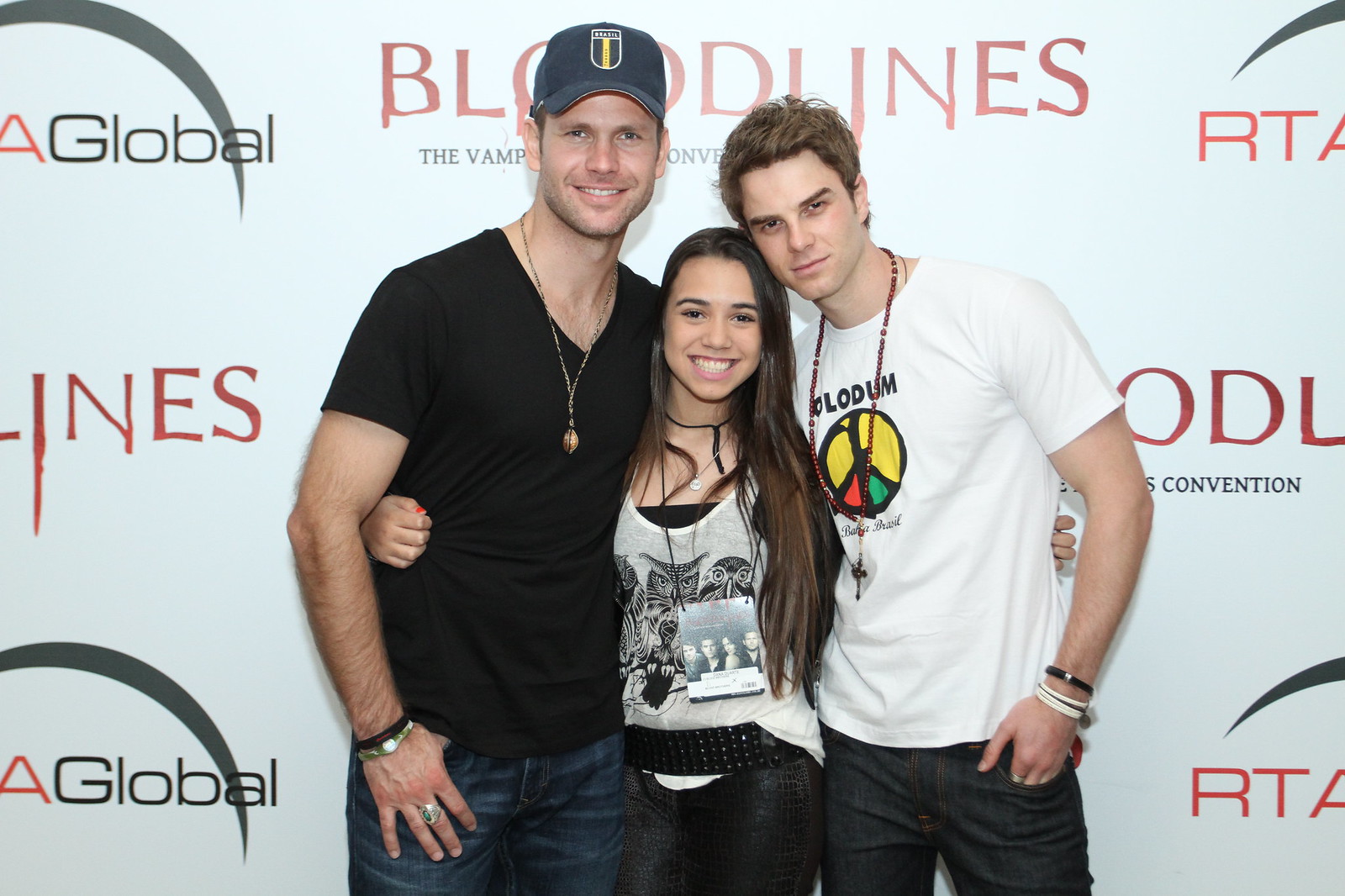This photograph captures three individuals, likely at a premiere event, posed in front of a branded backdrop, commonly used for such occasions. The backdrop is light blue with various sponsors' logos, prominently including "Bloodlines: The Vampire Convention" in bold red letters with smaller black text and "RTA Global" in red and black lettering with a black arch motif.

The group comprises a taller man on the left in a black t-shirt, blue jeans, a blue baseball cap featuring "Brazil," and a necklace. In the middle stands a shorter woman, wearing a white t-shirt with an owl design, a black shirt underneath, and dark jeans or black leather leggings. She also sports a necklace. To her right is another man, taller than the woman but shorter than the first man, donning a white t-shirt with a colorful peace sign, dark blue jeans, a mixture of white and dark bracelets, and a necklace.

The setting suggests they are attending a high-profile event linked to a vampire-themed series or convention, indicated by the "Bloodlines" branding in the background.